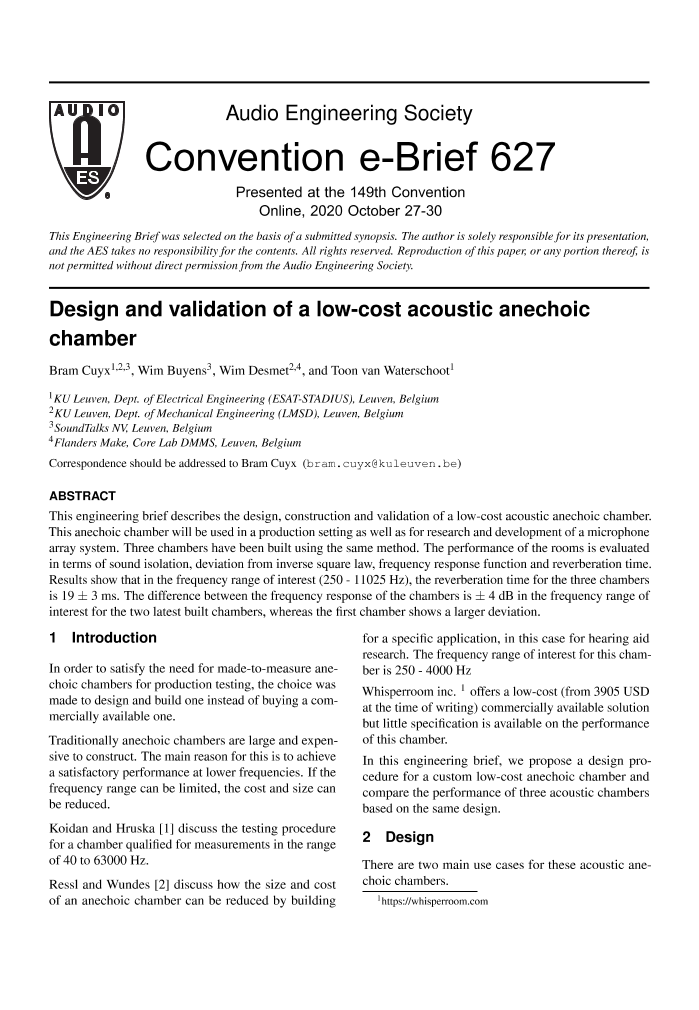The image depicts a scan of a document from the Audio Engineering Society, featuring their logo in the shape of a shield on the upper left corner, labeled with "Audio" on top, "A" in the center, and "ES" beneath it. The header at the top of the page reads "Audio Engineering Society," followed by the subheading "Convention E-Brief 627," and indicates that it was presented at the 149th Convention Online 2020 from October 27th to 30th. The main title of the document is "Design and Validation of a Low-Cost Acoustic Anechoic Chamber." An abstract paragraph spans the width of the page below the title, summarizing the paper, which includes contributions from authors Bram Kiox, Wim Bienz, Wim Dessit, and Thun Van Waterschutz. The document then continues into a structured layout with headings such as "Introduction" and "Design," followed by detailed paragraphs and additional footnotes. The paper is subject to copyright by the Audio Engineering Society, and reproduction without direct permission is prohibited.